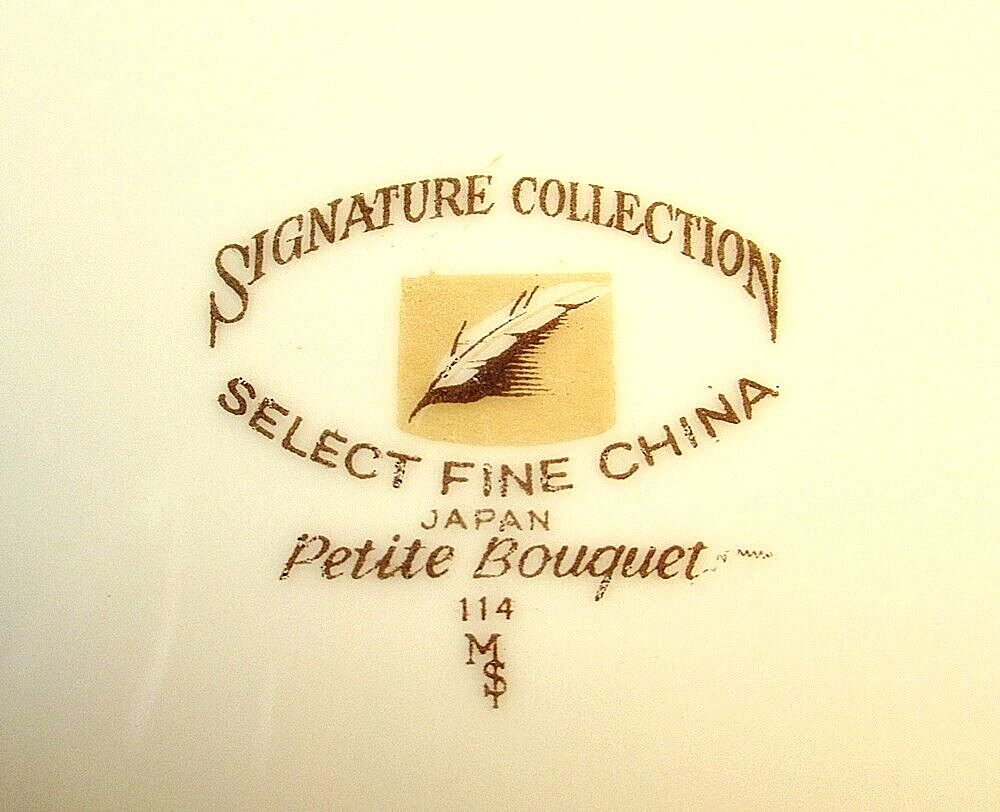The image depicts a finely detailed logo stamped on a piece of fine china. The background is a creamy bone color typical of high-quality porcelain. At the center of the image, in a very dark brown, all-caps font, the words "SIGNATURE COLLECTION" encircle the top of a prominently placed yellowish-brown square. Inside this square, a delicate cream-colored feather, casting a dark brown shadow, is positioned diagonally from the bottom left to the top right corner. Below the feather, also in the same dark brown, all-caps font, it reads "SELECT FINE CHINA," followed by "JAPAN" in even larger all-caps. Beneath these words, in an elegant cursive font, it says "PETITE BOUQUET," with the number "114" underneath. At the very bottom, a distinctive logo featuring the intertwined letters "MS" is present, with the right leg of the 'M' extending downward, intersecting the 'S'. This logo and inscription are typically found on the underside of fine china pieces, indicating the maker and the collection.